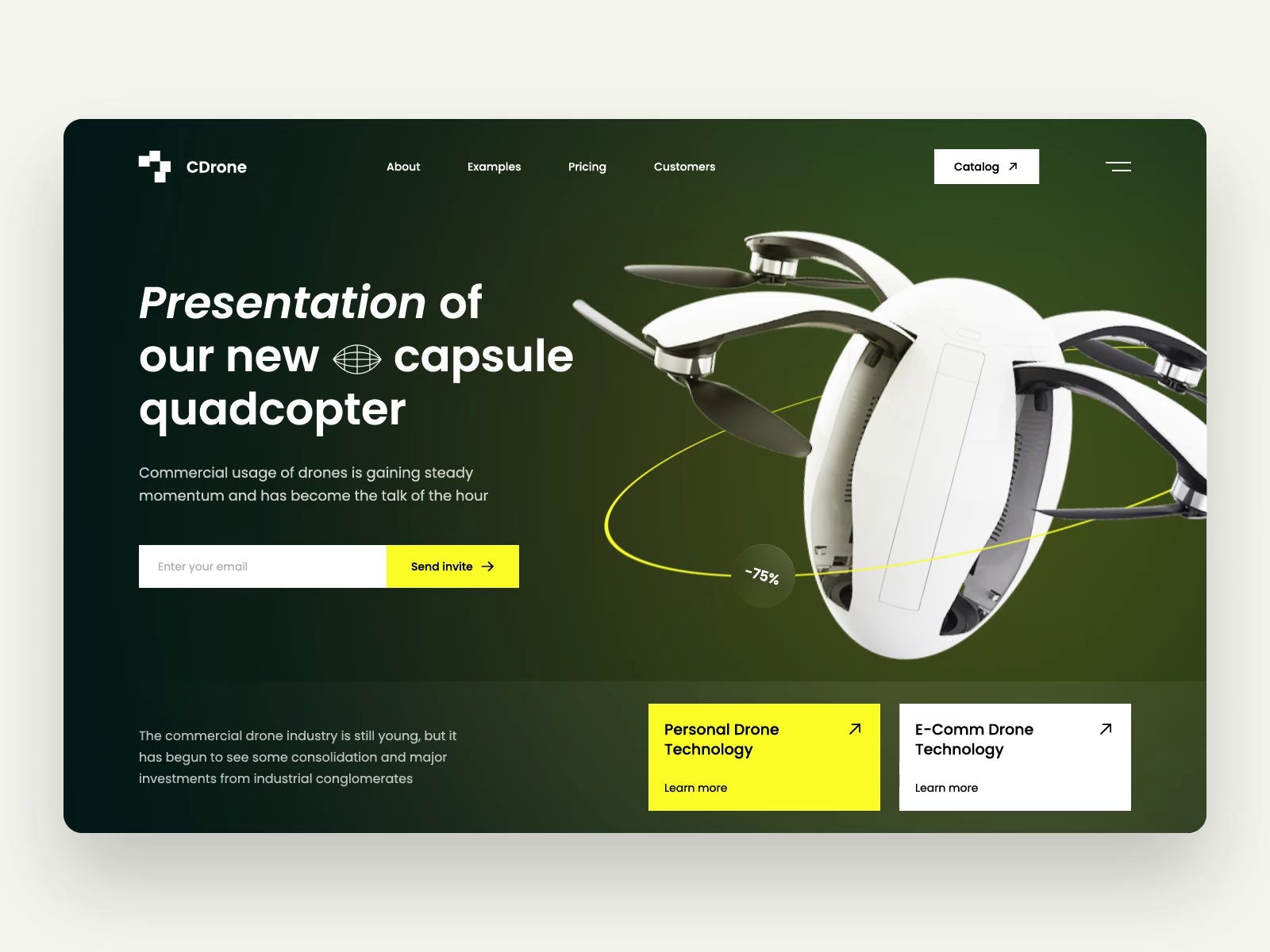**Detailed Caption for the Website Screenshot:**

The screenshot showcases a sleek, dark-themed website titled "C Drone." In the top-left corner, the logo comprises four white boxes arranged to form an abstract shape reminiscent of the top half of a question mark. To the right of the logo, text links for "About," "Examples," "Pricing," and "Customers" are displayed in clean, white typography. Further to the right, in the top-right corner, a button labeled "Catalog" offers access to the product catalog. Adjacent to this button, two horizontal bars suggest the presence of a drop-down menu.

The central focus of the page features a prominent headline in bright white text on the left side: "Presentation of Our New Football Capsule Quadcopter." Below the headline, a subtext in white reads, "Commercial usage of drones is gaining steady momentum and has become the talk of the hour." There is also an input field inviting users to enter their name and send an invite, indicating that access to the site may be invite-only.

On the right side of the main content area, a visual representation of the innovative football-shaped quadcopter is displayed. This drone resembles a football, with parts extending upward to form wings. Beneath this image, a yellow-highlighted section reads "Personal Drone Technology" with a "Learn More" arrow, suggesting a submenu or additional information. Directly to the right of this section, a clickable white box titled "EECOM Drone Technology" offers a link to another webpage for more details.

Overall, the website's dark background contrasts sharply with the bright white and yellow elements, ensuring that the key information and interactive features stand out prominently.